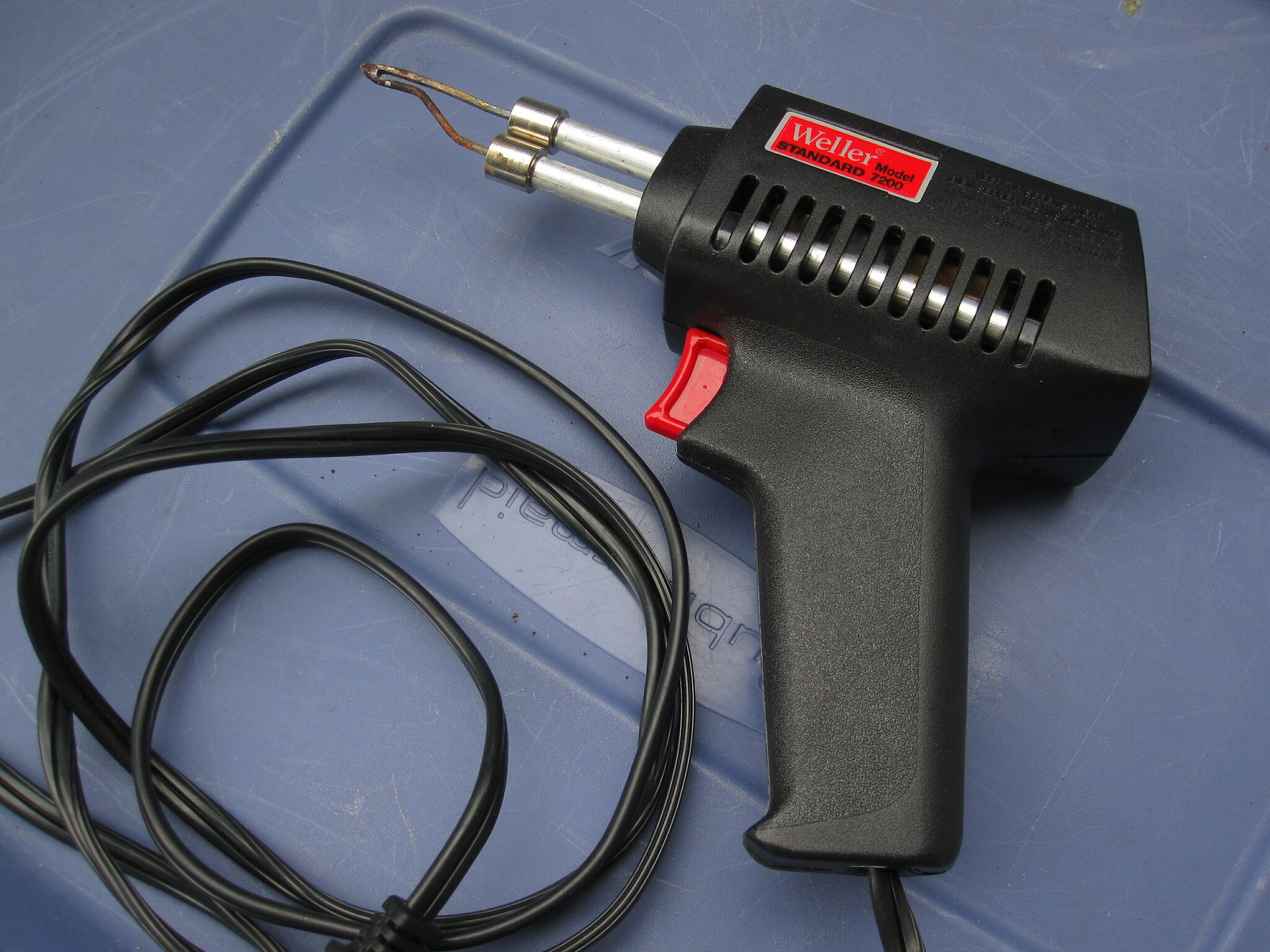The image displays a black soldering gun produced by Weller, prominently featuring a red rectangular logo sticker. This logo includes the silver text "Weller" and the words "Standard Model 7200" in black. The soldering gun has a distinct red trigger and is equipped with two white rods extending from the front, each terminating in metal tips connected by a rusted, inverted U-shaped metal coil. An electrical cord, coiled neatly into circles, is attached to the gun. The entire setup is positioned on the blue plastic lid of a Rubbermaid storage tote, with the word 'Rubbermaid' appearing upside down in the background.